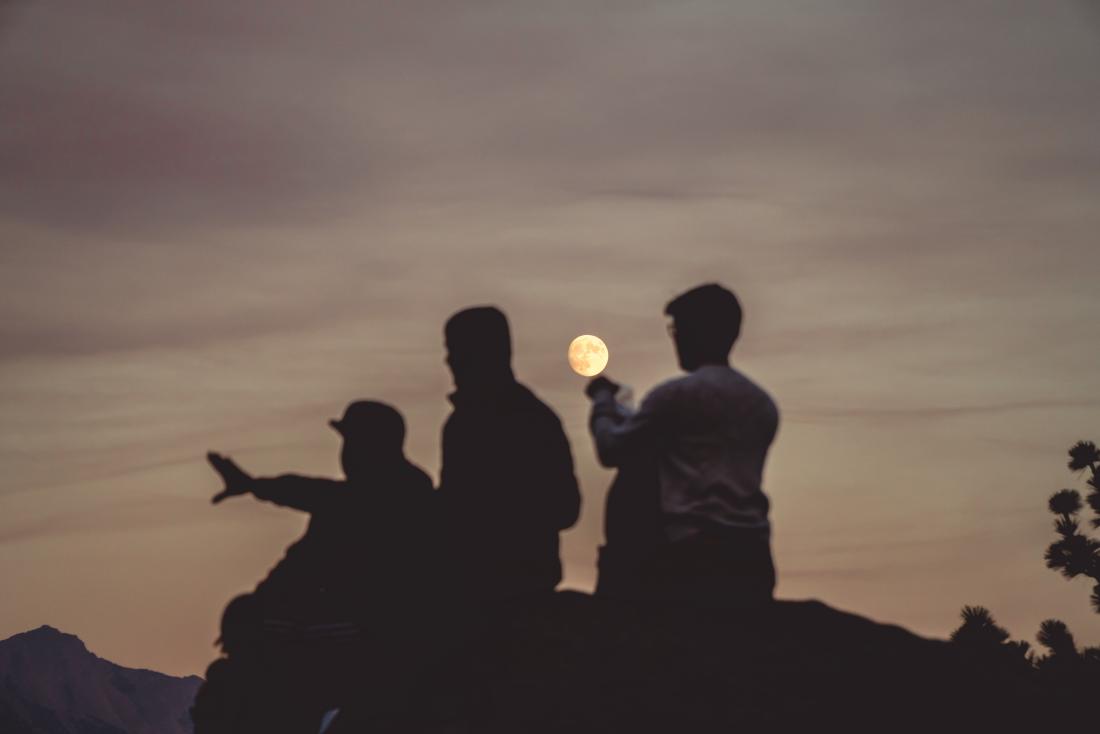The photograph captures a poignant moment on a mountaintop at dusk, showcasing a serene landscape beneath a brooding, gray sky. Three men, who appear to be in their early 30s, are seated on a rocky outcrop, gazing at the horizon. The man in the middle is distinguishable by his white long-sleeve sweatshirt and hat; he extends his hands outward, making it appear as though he's holding the small, crystal-clear, yellow-toned moon that hovers just above his hands. The other two men, to his left, are shrouded in shadow, adding to the dramatic contrast of the scene. In the background, on the right side, a dense forest of black trees frames the image, while to the left, a rugged mountain range stretches out. The enchanted setting, with its blend of natural elements and human silhouettes, evokes a tranquil and reflective mood.